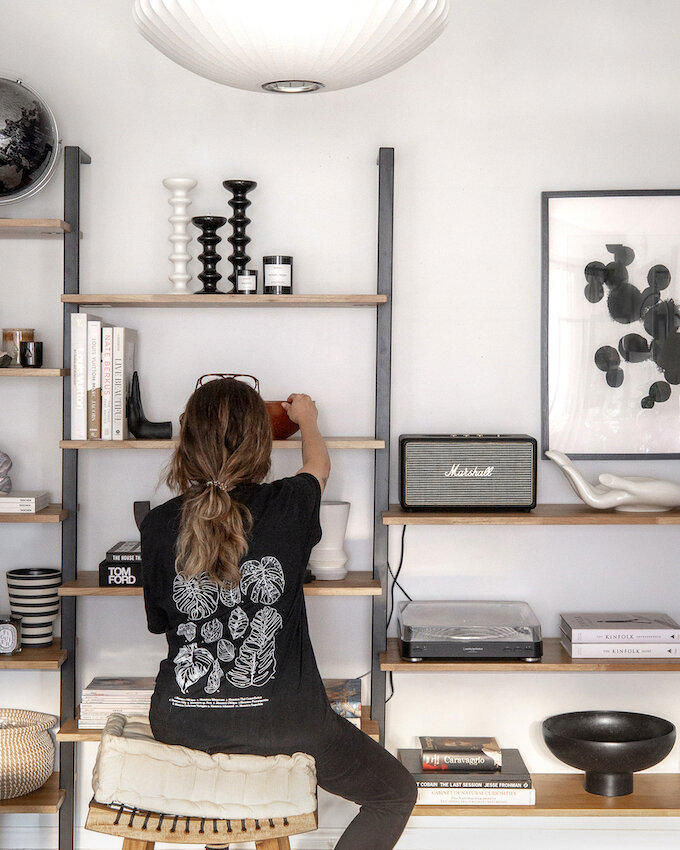In this detailed photograph, a young woman is seated with her back towards the camera on a backless wooden chair with a white cushion. She is organizing items on a multi-tiered shelf unit in front of her. The woman, dressed in a black shirt adorned with black-and-white plant drawings and black pants, has long brown hair tied back in a ponytail. Her eyeglasses are perched on her forehead as she reaches out with her right hand, touching a bowl on the second shelf from the top.

The shelf unit itself is filled with various items of interest. On the top shelf, there are candle holders of different sizes, along with candles – some black and some white. Additionally, there's a globe situated on the top left and a lighting fixture above the area, featuring a rounded glass design. Below, we see the shelf unit holding a curated assortment of books including Tom Ford photography, a small amp with the brand name Marshall visible, and a turntable. More knickknacks are arranged on the other shelves, including a radio, a small statue of a hand, and what appears to be a tin-type bowl on the bottom shelf.

To the right of the shelf unit, there is another wall display with multiple small shelves filled with plaques, baskets, glasses, and other decorative items. A framed painting featuring black dots on a white background is also visible on the right side of the scene. The overall setting of the room is well-lit, providing a clear view of the orderly and aesthetically pleasing arrangement.